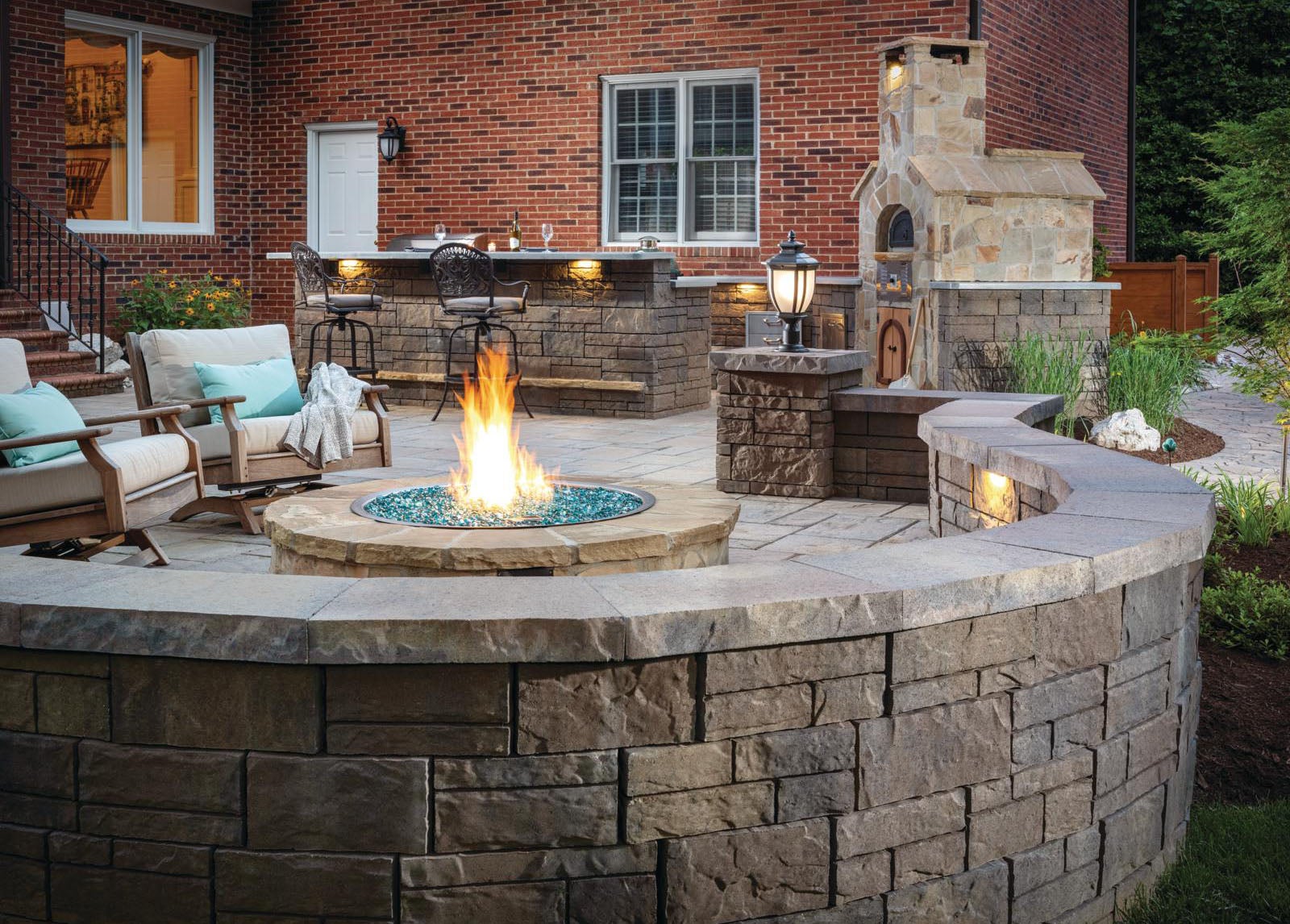The image is a highly realistic photograph, or an exceptionally detailed drawing, showcasing a meticulously designed backyard patio area. In the far background, a black and brown brick and mortar house stands with two windows and a door featuring a light fixture above. Moving closer, there's a prominent stone or brick island table flanked by two chairs with lighting installed underneath, giving it a cozy, ambient feel. On the right, you find a substantial outdoor pizza oven, which shares the same brick aesthetic as the island. 

Prominently in the foreground, there's a circular stone fire pit encircled by a low, curved brick wall about a foot and a half tall with recessed lighting. The fire pit itself features light blue stones and an artificial-looking orange fire, giving off the peculiar appearance of having ice where the embers should be. To the left of the fire pit, two wide, comfortable armchairs resembling Lazy Boys or large computer chairs are placed, each adorned with thick gray cushions and additional blue seat toppers. Behind these chairs, a set of stairs leads upward, presumably towards the house. 

Additionally, to the right of the fire pit, there is a small garden area with a few little trees, a decorative fence, and a pathway leading toward the circular fire pit space. The entire style of the backyard is very modern, with a strong emphasis on stone and brick materials, creating a sophisticated and inviting outdoor living area.